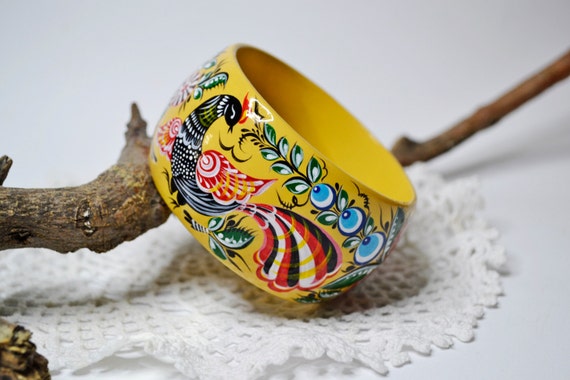The image depicts a yellow ceramic object, possibly a bracelet or napkin ring, with intricate painted designs. Prominently featured is a black-bodied rooster or peacock with red and white wings and a red crown, surrounded by either red, white, and black plumage or green leaves. The object is tilted on its side, revealing its curved form, and is set against a thick brown tree branch that tapers into the background. This entire scene is displayed on a delicate, crocheted white lace doily, adding an intricate, textured backdrop. Additionally, there is a plant with white and blue blossoms visible in the composition, enhancing the overall decorative appeal.